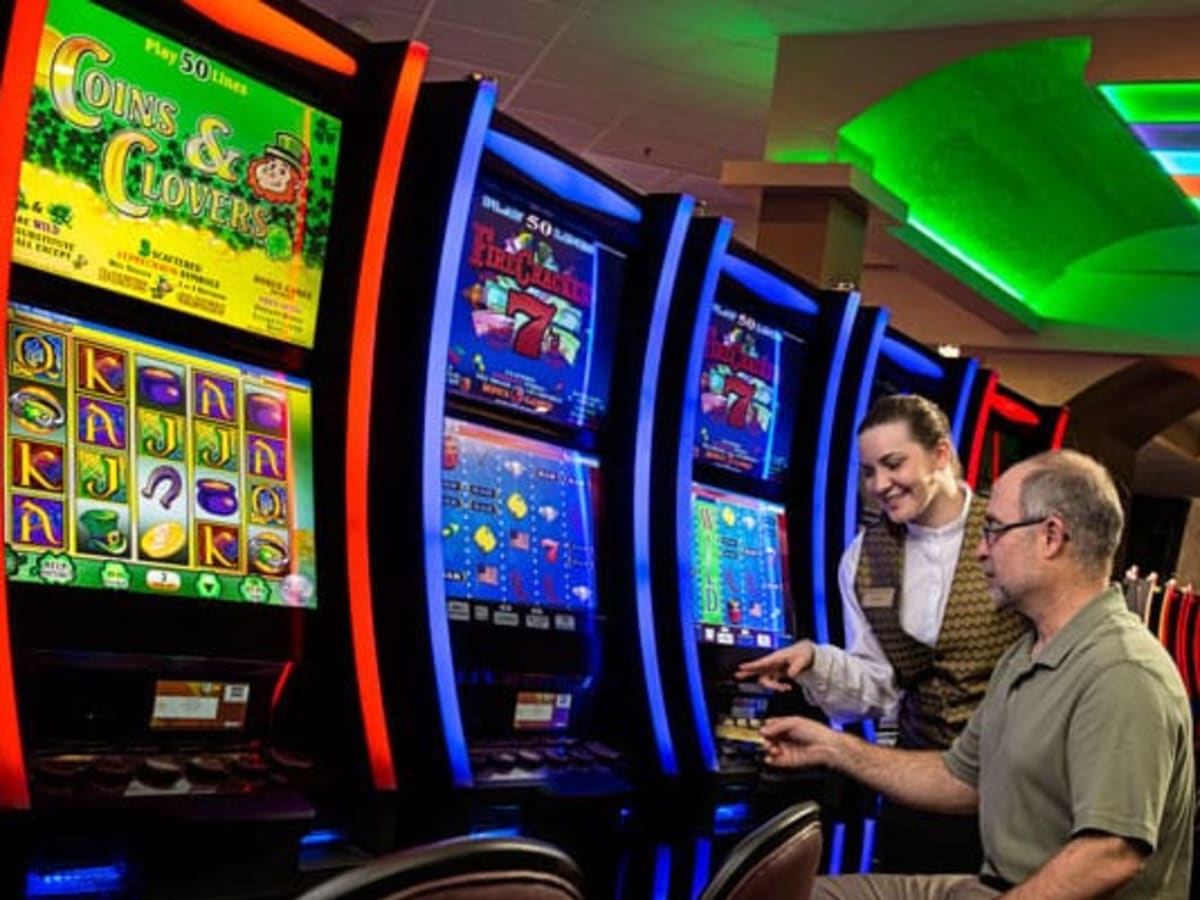The image captures a lively casino scene with a row of vibrant slot machines. On the left, there is a red "Coins and Clovers" machine, adorned with a leprechaun mascot, highlighting its charming Irish theme. Next to it are two identical blue "Firecracker 7" machines, each designed with five different betting lines. On the far right, a partially visible red machine can be seen, adding to the colorful array. In front of one of the "Firecracker 7" machines, a woman who appears to be a casino employee is pointing out details to a man seated at the machine. The man is dressed in a light olive green polo shirt, intently focusing on the explanation. The casino ambiance is accentuated by a ceiling with an arch, illuminated by a green light that adds to the visual appeal of the setting.